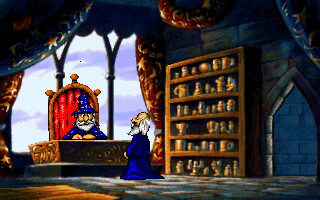In this vibrant fantasy cartoon image, a mystical scene unfolds within the confines of a medieval-style stone castle. At the center, a grand desk is riveted by a majestic, red, and gold-outlined chair. Sitting regally on the chair is an elderly wizard, distinguished by his flowing white beard and a pointed blue wizard hat. His light skin contrasts against the decadent red upholstery. Behind him, through an arched window, the sky appears a dreamy, cloudy blue, adding a celestial backdrop to the enchanting setting.

To the right of the scene stands a bookshelf, brimming with a plethora of ancient tomes and curiosities. Adjacent to it, another elder wizard makes his presence known. Unlike his seated counterpart, this wizard sports a tuft of white hair at the back of his head and a full white beard, but forgoes a hat. He is clad in a blue robe that closely mirrors the attire of the seated wizard. Further enhancing the magical atmosphere are the luxurious blue and gold drapes that elegantly cascade around the stone walls of the castle chamber, infusing the scene with an air of opulence and mystery.